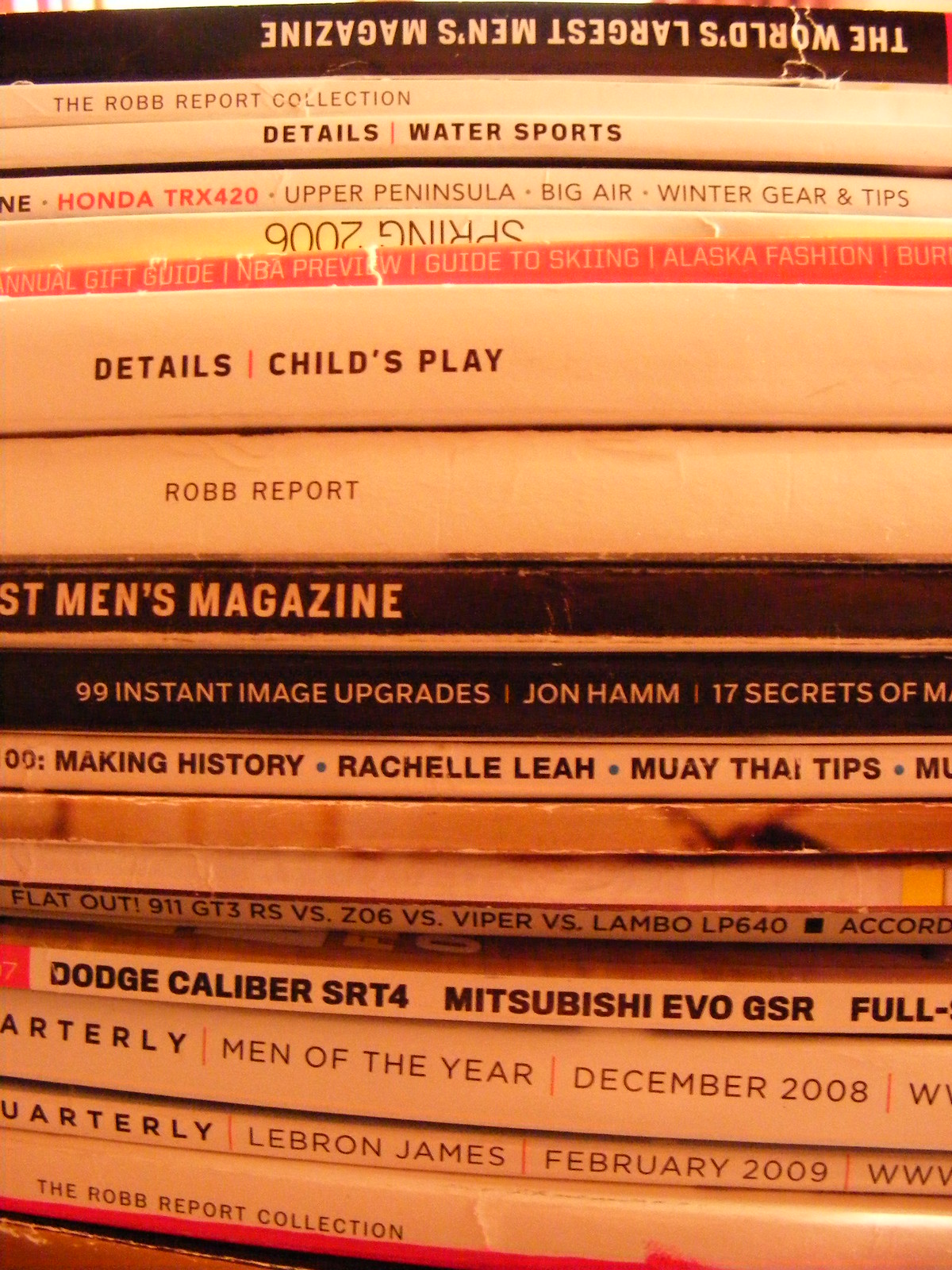The image is a close-up shot of several magazines stacked on top of each other, with their spines facing the camera. The scene has a brownish tint caused by an orange-hued light source casting a shadow over the magazines. These publications appear weathered and worn, suggesting they are from around 2008-2009. Among the visible titles are the Robb Report Collection, Man of the Year (December 2008), a magazine featuring a Dodge Caliber and Mitsubishi, Flat Out (with a feature on Viper versus Lambo), Rachel Lee Making History, 99 Instant Image Upgrades, and another Robb Report detailing Child's Play. Some of the spines show partial titles, such as a men's magazine and another issue of the Robb Report mentioning LeBron James (February 2009). The magazines vary in thickness and cover styles, including black covers with white letters and white covers with red or black letters, indicating a diverse collection that includes sports and car magazines. The close-up nature of the image restricts the view to just the stack, with no background or room detail visible.